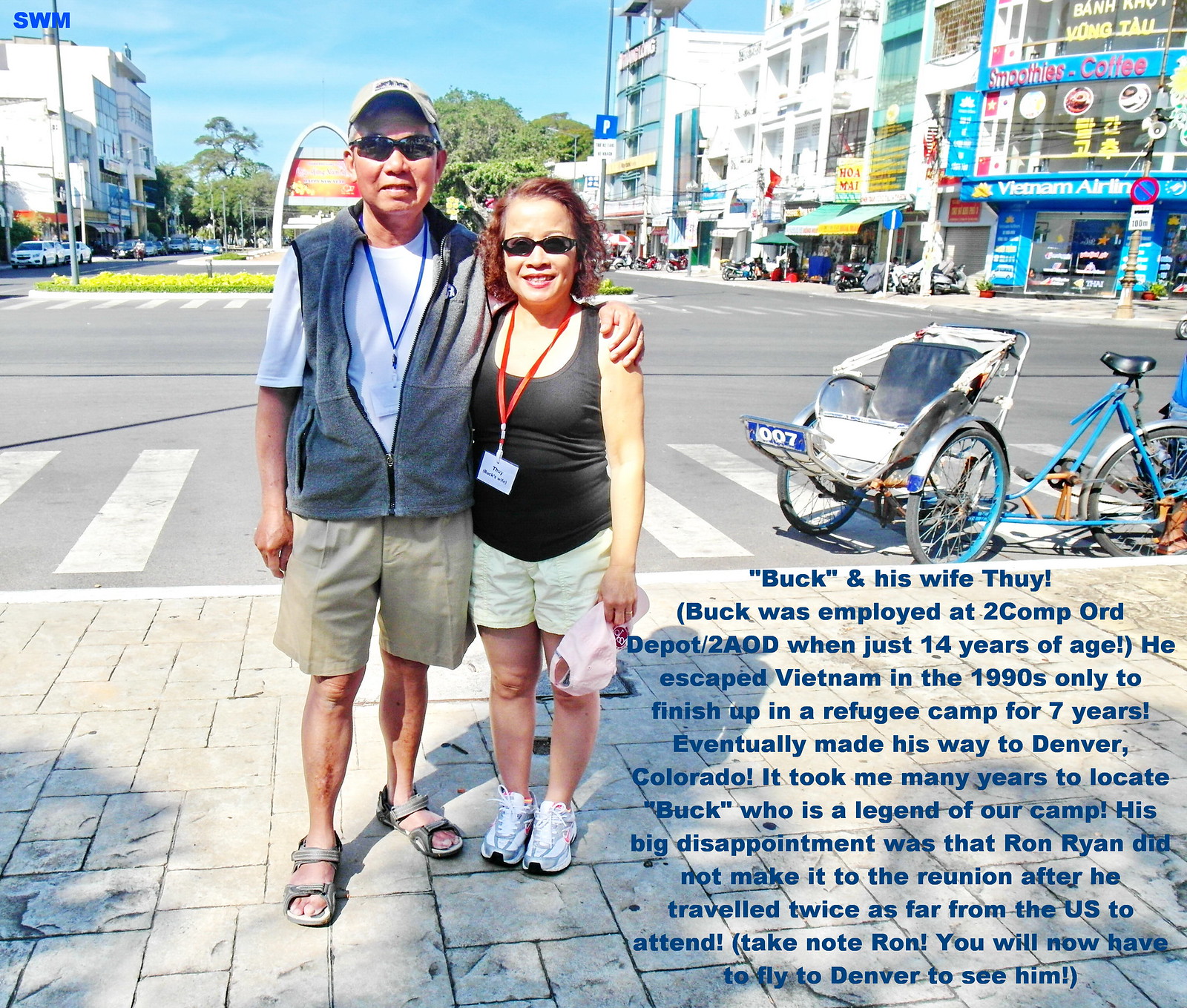The photograph captures a vivid street scene in Vietnam, featuring a man and a woman, identified as Buck and his wife Thuy. Both are wearing sunglasses and lanyards—Buck's is blue and Thuy's is red — which hold placards resembling press passes. Buck is dressed in a white cap, sunglasses, a gray vest over a white shirt, and khaki shorts. Thuy stands on his right, sporting a black sleeveless shirt, yellow shorts, tennis shoes, and holding a pink hat. She has curly red hair and is about a head shorter than Buck. To their right, the bustling street is lined with several stores and awnings under which people are milling about. Also on the right side of the image is a bicycle with a passenger wagon attached. In the lower right corner, text reads: "Buck and his wife Thuy. Buck was employed at 2 Comp Ward Depot, 2 AOD, when just 14 years old. He escaped Vietnam in the 1990s, only to end up in a refugee camp for seven years before eventually making his way to Denver, Colorado. It took many years to locate Buck, who is a legend of our camp. His major disappointment was that Ron Ryan did not make it to the reunion despite traveling twice as far from the U.S. to attend. Take note, Ronnie, you will now have to fly to Denver to see him." The photo captures a slice of life and a poignant story of resilience and reunion amidst a vibrant Vietnamese street.